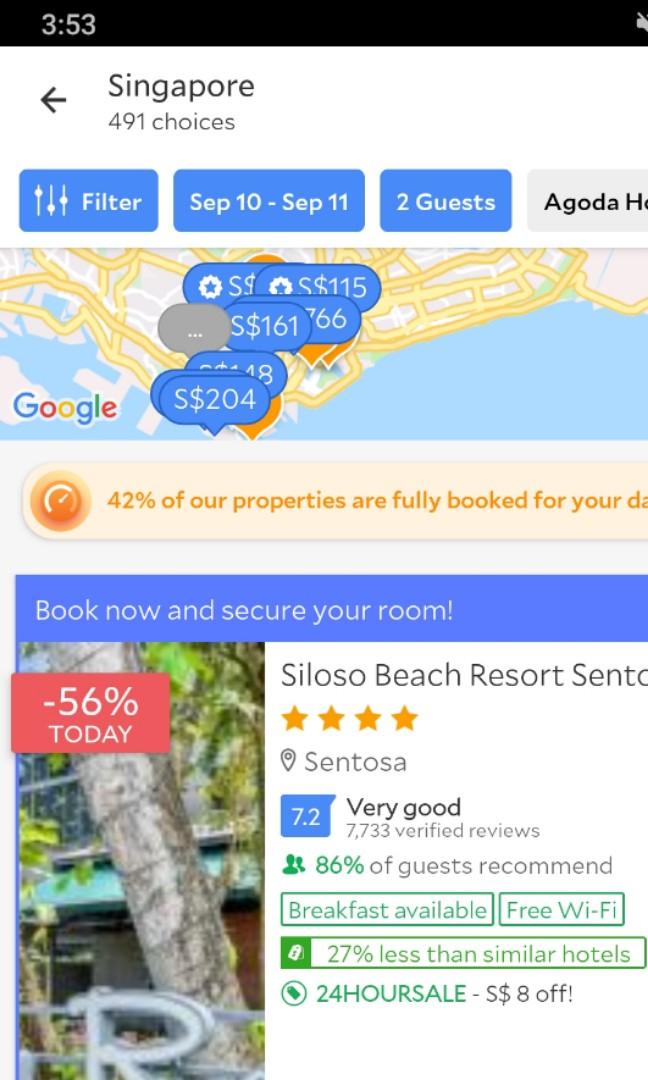Screenshot Overview: Singapore Hotel Search Results

- Time Displayed: 3:53
- Location: Singapore
- Total Options: 491 choices
- Filters Applied: 
  - Dates: September 10th to September 11th
  - Number of Guests: 2
  
Filter Buttons Present

Google Map Overview:
- Displaying local resorts and their pricing

Availability Notice:
- "42% of our properties are fully booked for your dates."

Search Result Highlight:
1. **Celso Beach Resort Sentosa**
   - Located in Sentosa area
   - Rating: 4 stars
   - Customer Satisfaction: Very good, with a score of 7.2
   - Verified Reviews: 7,733
   - Guest Recommendation: 86% recommend
   - Amenities: Breakfast available, free Wi-Fi
   - Price Comparison: 27% less than similar hotels
   - Limited Offer: 24-hour sale, with an additional $8 off
   - Special Discount Banner: 56% off if booked today